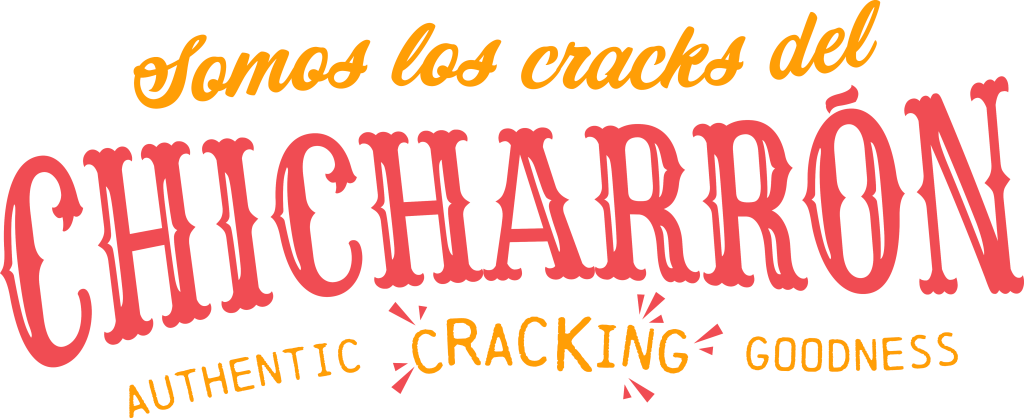The image appears to be an advertisement for a food product, prominently featuring the word "CHICHARRÓN" in large, bold, red, all-capital letters, with a tilde above the last "O", arranged in a curved line across the center. Above this, in bright yellow text, it says "Simoes, Loss, Cracks, Dell." Below "CHICHARRÓN", in the same bright yellow, curved text, are the words "Authentic Cracking Goodness," with "Cracking" having disproportionately larger letters (R, C, and K) and small red streaks or motion indicators to make it appear as if it is erupting or popping out. All of this text stands out against a pure white background.